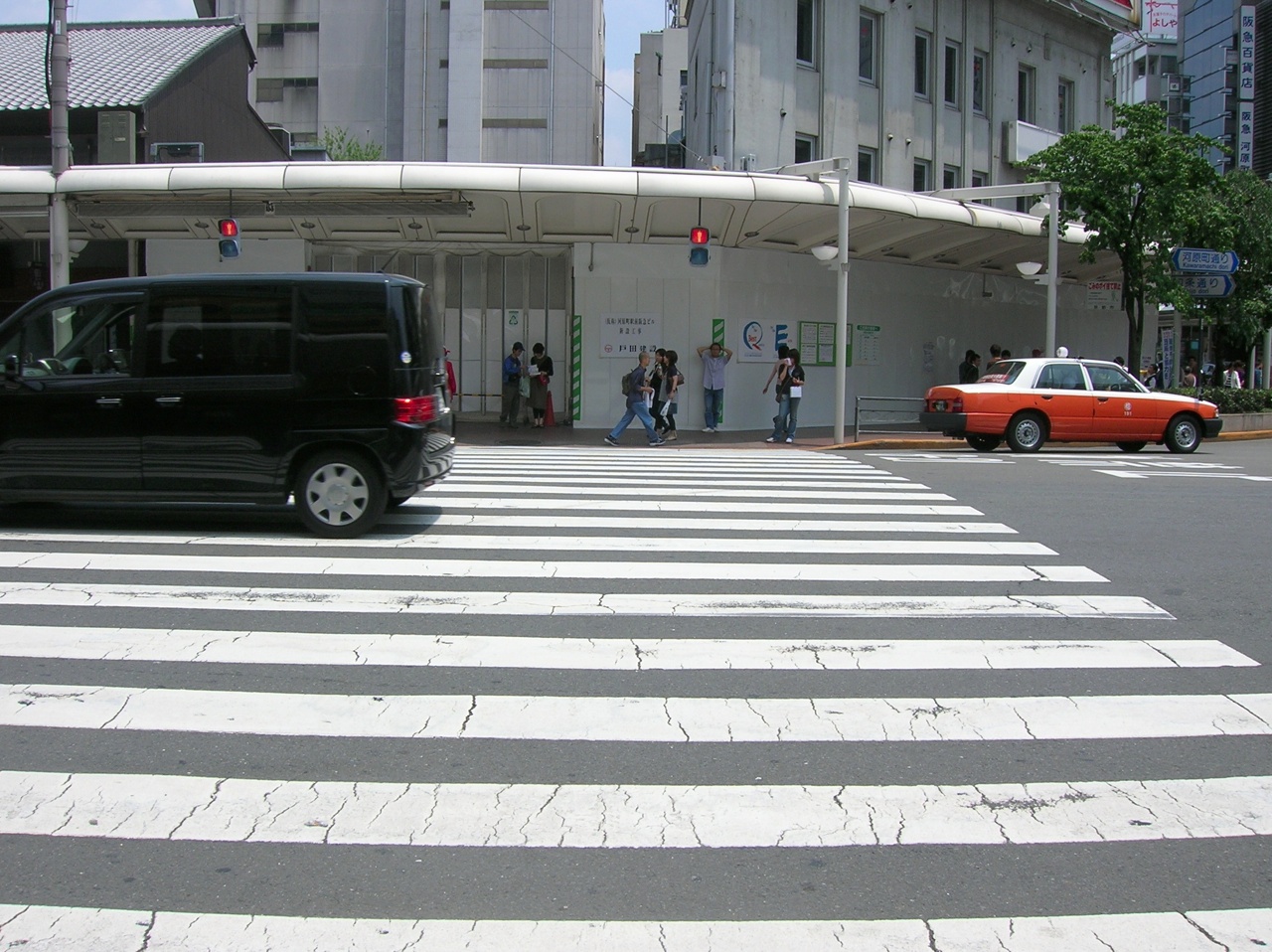The photograph captures a bustling city corner from the perspective of someone about to step onto a wide white crosswalk that spans almost the entire width of the frame. On the left, a black van is partially out of the frame, heading left. To the right, a red and white taxi approaches, moving towards the right side of the image. Across the street, a group of people mill about under a large white awning, which extends from a round white building that appears to be either multi-story or in front of taller white buildings. The scene includes a mix of architectural elements, with the white building featuring posters and papers on its wall and a darker gray building visible on the upper right. Also noticeable are some rectangles with dark and light green stripes and a tree on the far right. The street itself shows signs of wear, with visible cracks in the pavement, set against the backdrop of tall, slim buildings.